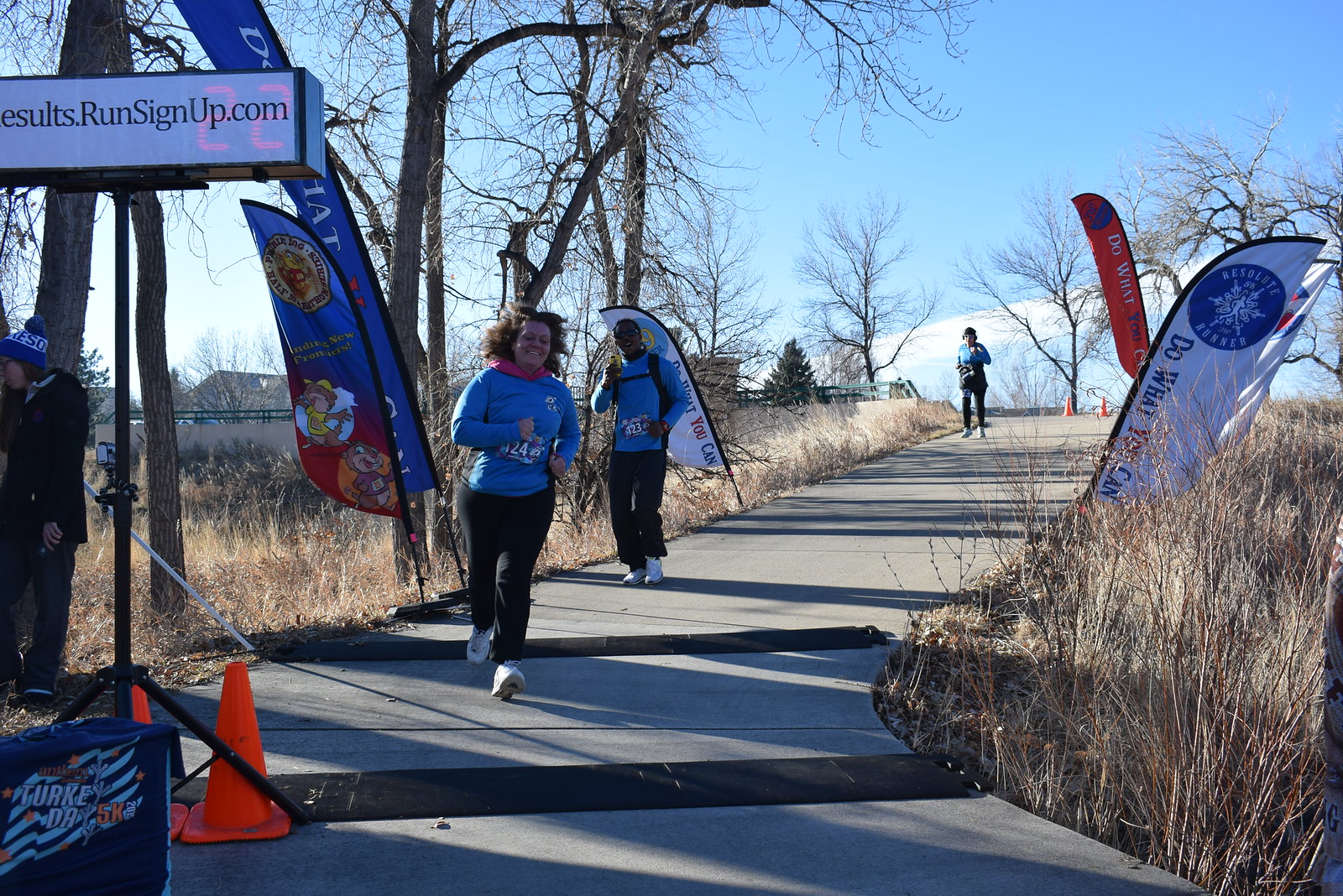In this photograph, a trio of runners is captured on a paved track, which cuts through a field of tall, hay-like grass. The scene is dominated by leafless trees, indicating it is winter. The runners are participating in an official race, as evidenced by the bibs they wear; the leading female runner, looking confident and relaxed, sports bib number 124 and is smiling. Following her is a male runner, marked by bib number 123, who appears to be African-American. A third runner, also female with dark brown hair, trails further behind. 

The track is lined with various banners and signs, including blue and white banners on the left and red and white banners on the right, guiding the participants. A prominent sign reads "results.runsignup.com," and a blue table in the lower left corner is marked with "Turkey Day 5K" in white text, managed by a woman in a blue beanie and black attire. Cones are set up around the track, and the sky above is a bright, clear wintery blue. The overall atmosphere exudes a well-organized race event set against a stark, seasonal landscape.